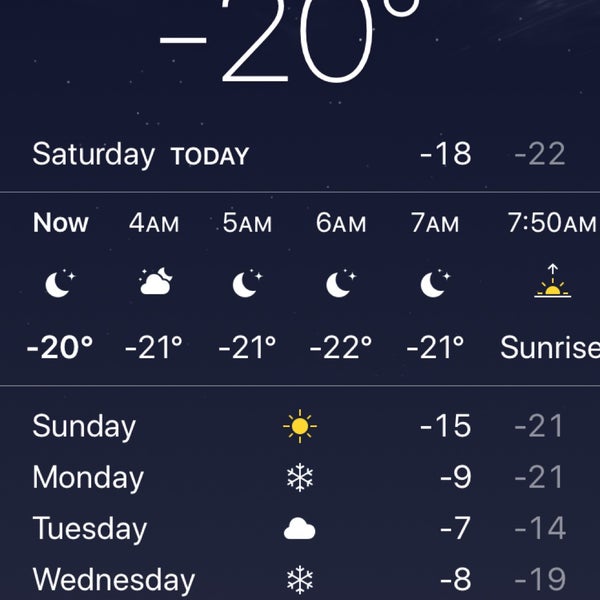This image captures a screenshot of a weather forecast displayed on a black background, with most of the text in white and some elements in gray. The top part of the screen is slightly cut off, but it clearly shows the current temperature of -20°C for Saturday and a projected high of -18°C with a low of -22°C (with the low temperature in gray). 

At the top, the display starts with the current weather status ("Now"), showing a moon icon partially obscured by clouds, indicating cloudy conditions and a temperature of -24°C. Over the next hours, the forecast shows:
- 4 a.m.: -24°C, cloudy
- 5 a.m.: -21°C
- 6 a.m.: -22°C
- 7 a.m.: -21°C
- 7:50 a.m.: Sunrise

On the left side, the forecast starts with the days of the week—Sunday, Monday, Tuesday, Wednesday (partially cut off)—each accompanied by icons representing weather conditions: a sun for clear weather, a snowflake for snowy weather, and a cloud for cloudy weather. Next to each day, the high temperatures are listed on the left and the low temperatures on the right.